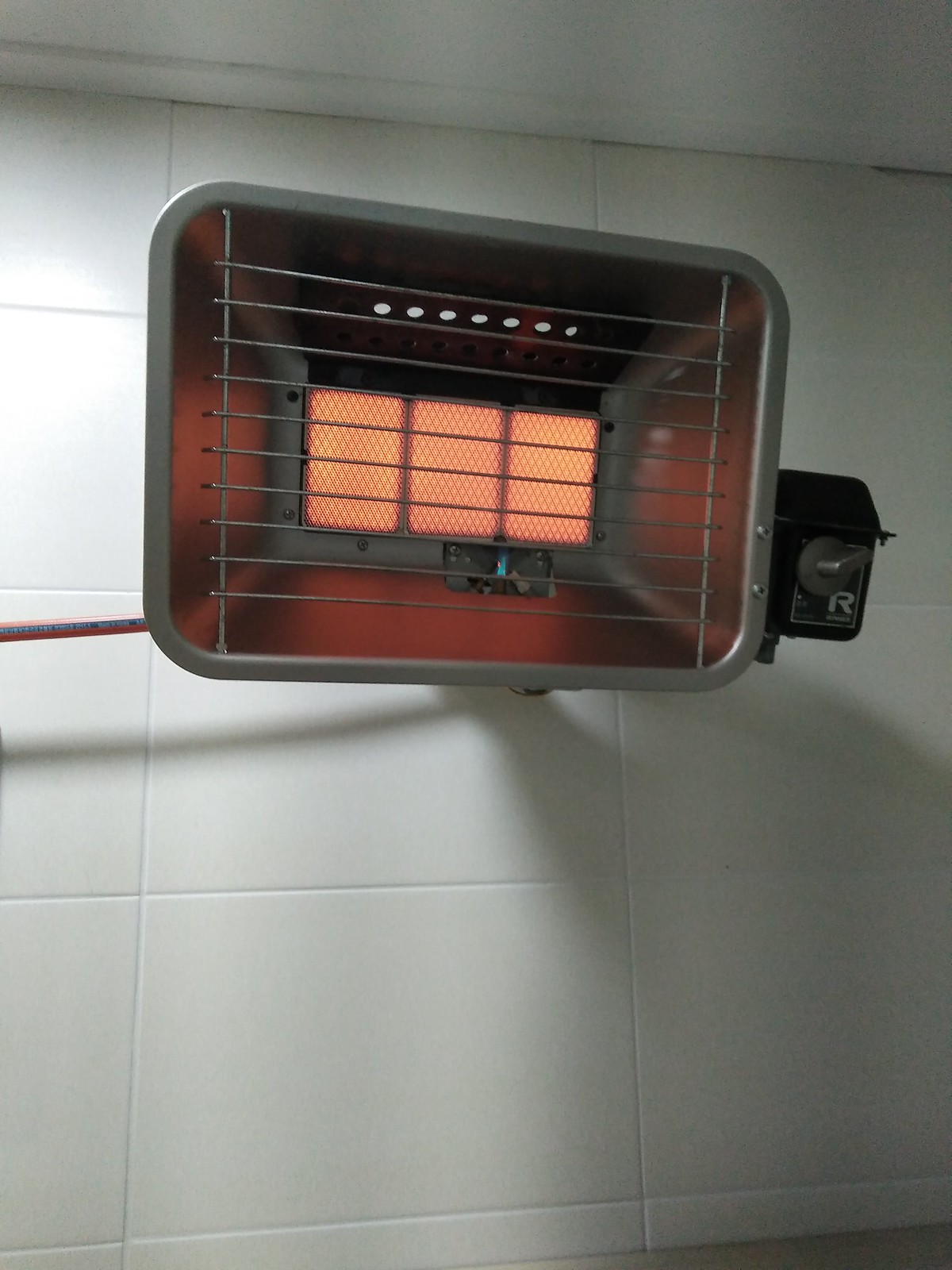The image showcases an up-close view of a wall-mounted electric heater affixed to a smooth, white tile wall. The heater, primarily rectangular with some square-like proportions, appears larger due to the close-up shot but is actually a compact unit. It is constructed from metal with a grill on the front to prevent direct contact with the internal heating element. The interior glows a vibrant orange-red, indicating that the heater is currently on. At the top of the heater, there are seven small, white teardrop-shaped elements visible. The right side features a black circular knob, turned to the right, signifying it's on. Below this knob is a black sticker adorned with a white "R" logo.